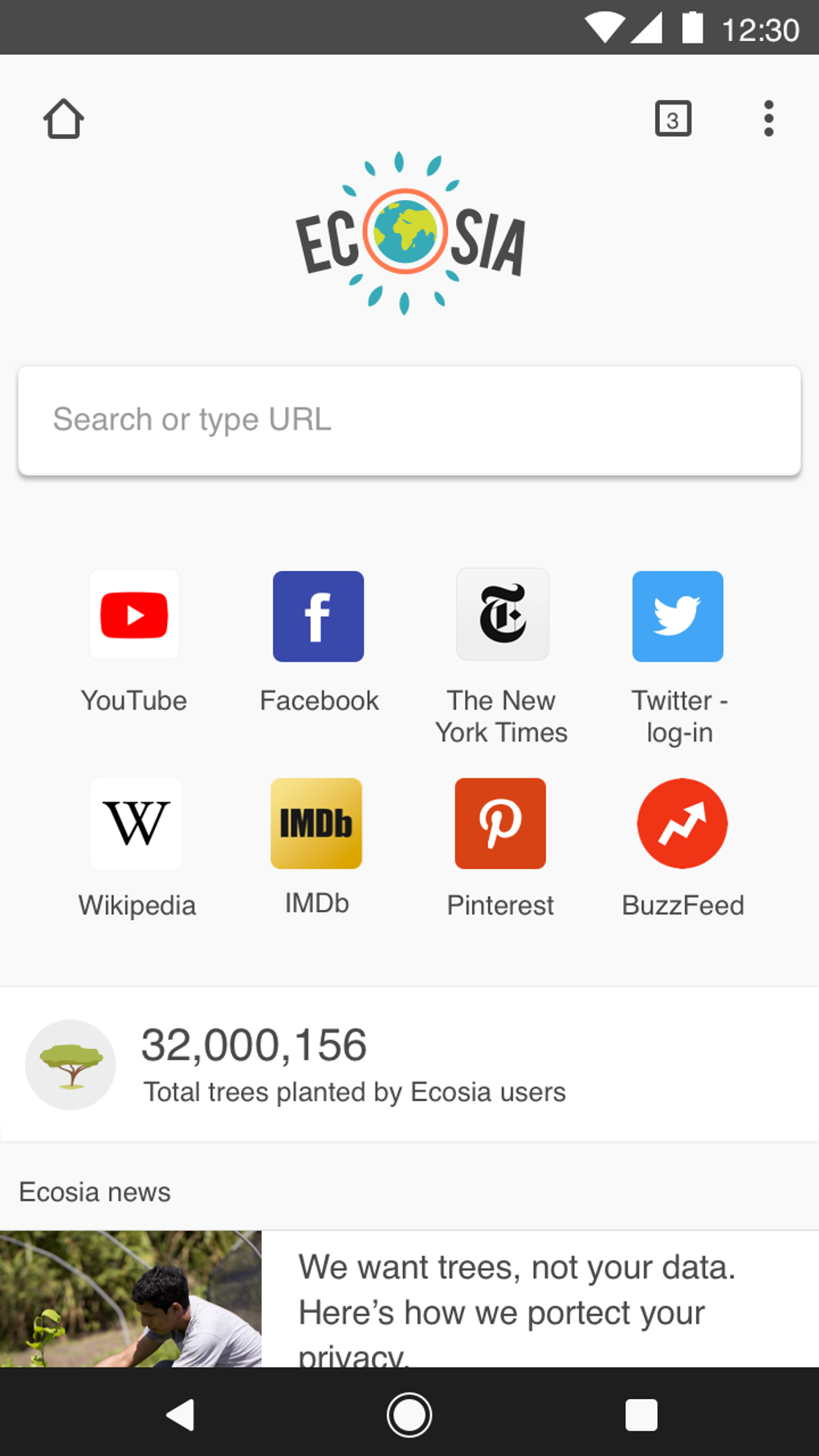Screenshot of an Android phone displaying the Ecosia web browser interface. The status bar at the top right shows blanked out Wi-Fi and cellular icons, with an unreadable battery level beside the time, 12:30. Below is the browser's search bar featuring the Ecosia logo—a cartoon world with a red circle and blue teardrops. The search input field reads, "Search or type URL."

Below the search bar is a series of popular website icons: a red play button for YouTube, Facebook's blue icon with a white "F," The New York Times' logo, Twitter's old blue bird icon, Wikipedia's stylized "W," IMDb's yellow icon with black text, Pinterest's red icon with a white cursive "P," and BuzzFeed's red circle with a white arrow. A prominent banner below these icons reads, "32,156,000 total trees planted by Ecosia users," highlighting the browser's eco-friendly mission.

At the bottom, a visual of someone planting a tree accompanies the text, "We want trees, not your data. Here's how we protect your privacy," with a typographical error in "protect." The standard Android navigation icons—back (triangle), home (circle), and recent apps (square)—are displayed at the very bottom of the screen.

Overall, this appears to be a screenshot highlighting the unique features of the Ecosia browser, designed for an environmentally conscious audience using an Android device.